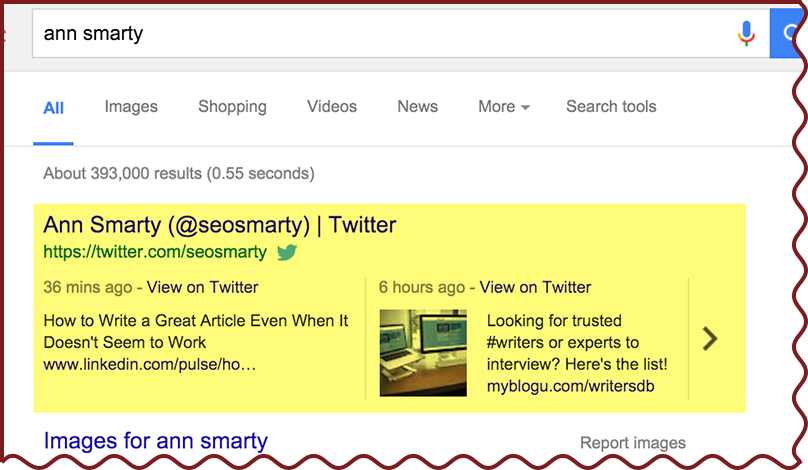Screenshot of a Google Search Results Page

This is a screenshot of a Google search results page taken on a desktop. The search query "Anne Smarty" is visible in the search bar, which also features a small microphone icon for voice search functionality. The primary navigation tabs—which include 'All', 'Images', 'Shopping', 'Videos', 'News', 'More', and 'Search tools'—are located just below the search bar.

The screenshot has irregular red markings: a red bar on the top right and squiggly red lines on the bottom and the right-hand side of the image. Google's search results indicate approximately 393,000 results found in 0.55 seconds.

Dominating the center of the page is a large, rectangular yellow box containing specific Twitter information about Anne Smarty, including:
- A Twitter handle: @SEOsmarty
- A timestamp: 36 minutes ago
- A snippet from a tweet: "How to write a great article even when it doesn't seem to work."
- A partial URL: "www.linkedin.com/.../Paul/...," trailing off without complete display.

Next to the large yellow box, additional information is displayed:
- A timestamp: "6 hours ago"
- Another snippet related to laptops: "Looking for trusted hashtag writers or experts to interview? Here's the list."
- A partial URL: unspecified website.

Finally, there's an option labeled "Report images" at the bottom of these results.